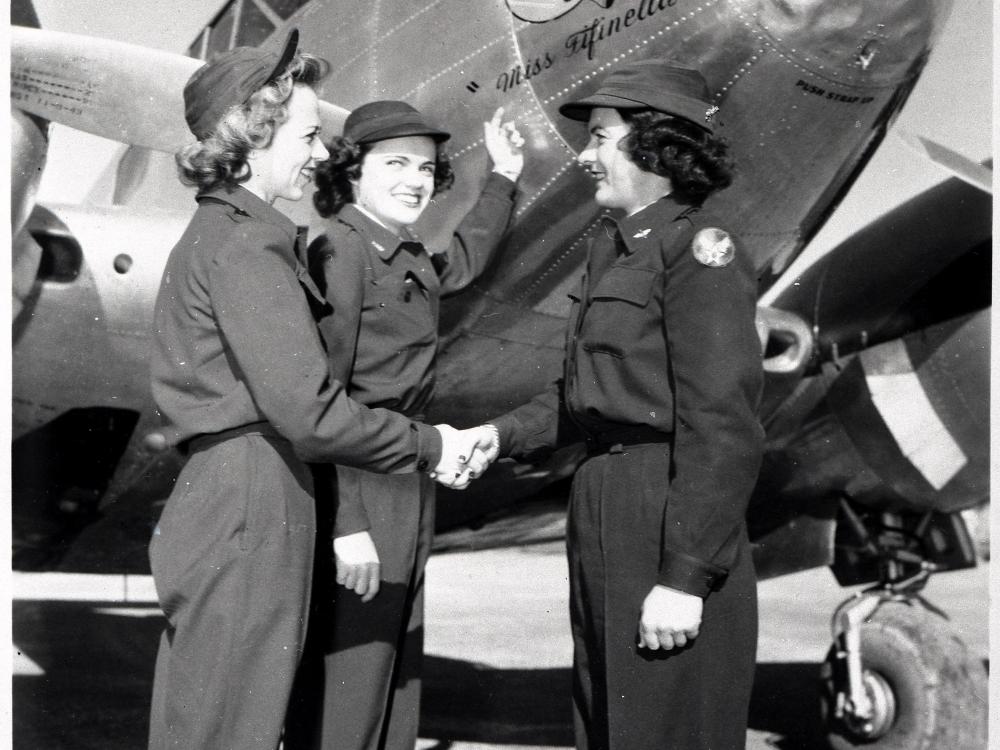This vintage black-and-white photograph depicts three photogenic women standing in front of what appears to be a World War II-era fighter plane. The plane's name, partially obscured, seems to read "Miss Fiffanetti" or something similar. The women are dressed in matching military-style uniforms comprising pants, jackets, and plain caps with a single brim. All three have short, curly hair, with the woman on the left having lighter hair and the other two having darker shades. The central woman smiles directly at the camera, while the two on either side are shaking hands and smiling at each other. The scene captures a sense of camaraderie and the vital role women played during the war, likely indicating that these women were among those who worked in factories or could be representing women pilots or military personnel.